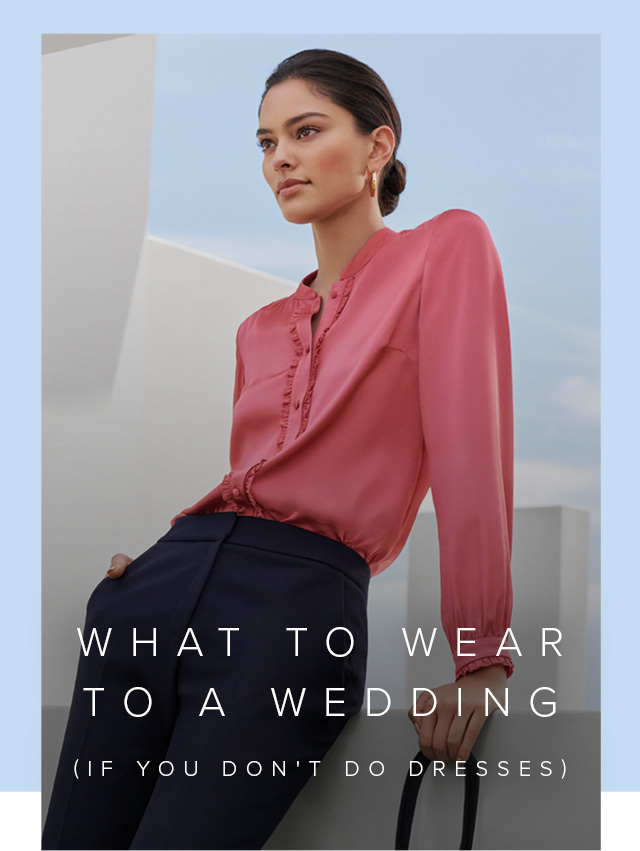The image appears to be part of a magazine article with an overlay text at the bottom reading: "What to wear to a wedding (if you don’t do dresses)." It depicts a stylish woman, likely of white or Latina descent, standing in front of an abstract background with a sky blue and white color scheme. She has dark brown hair pulled back into a bun and wears gold hoop earrings. She is dressed in a loose mauve rose-colored long-sleeved blouse with two frilly sections around the buttons, tucked into navy or black business-like pleated pants. She has her right hand in her pocket and appears to be holding a purse with her left hand, with only the strap visible. The woman's pose shows her looking off towards the viewer's left, adding to her poised and elegant demeanor.